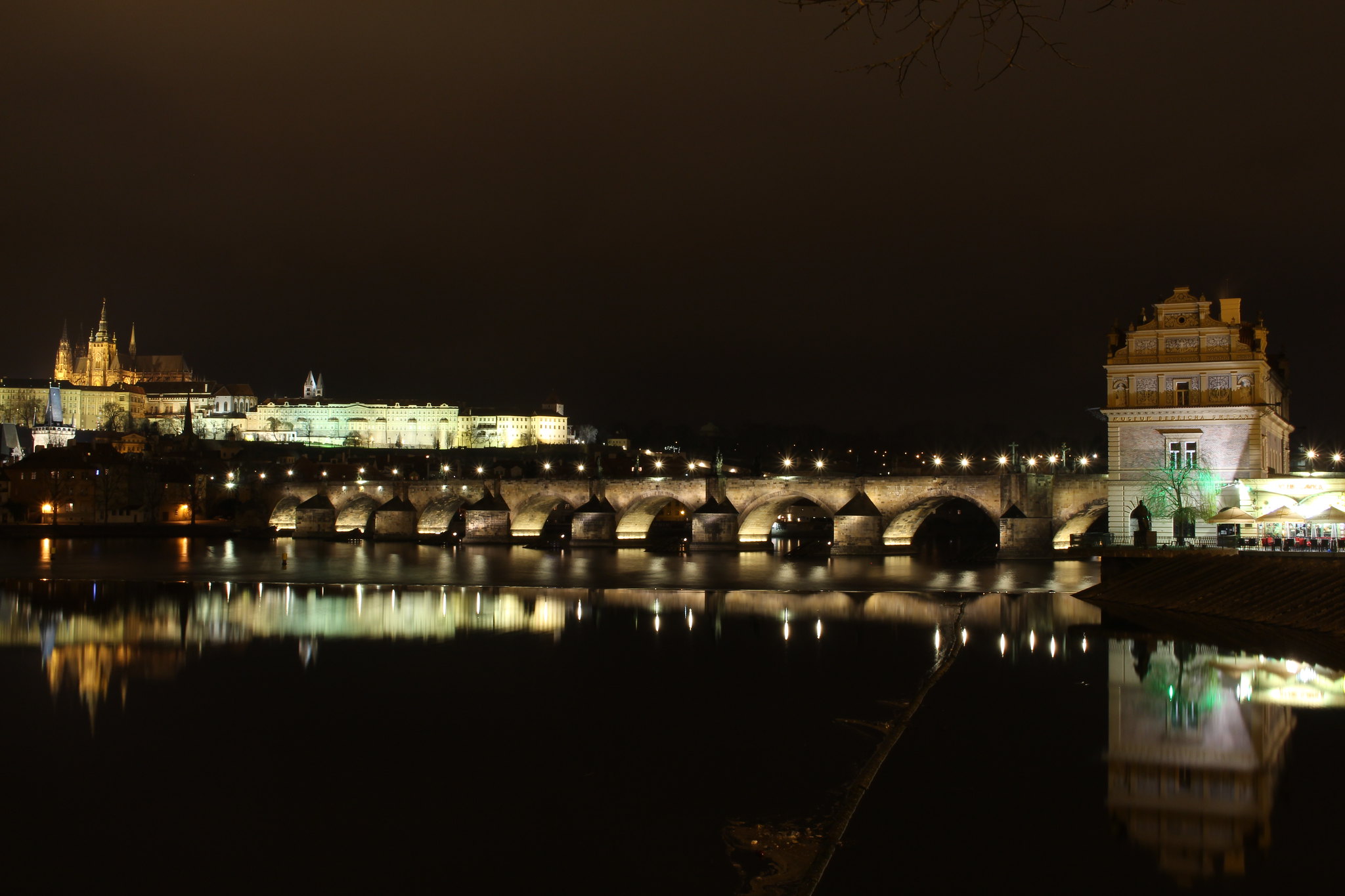A stunning nighttime photograph captures a picturesque scene likely set in Europe. In the foreground, a beautifully lit bridge with ornate railings spans a serene lake, offering a perfectly mirrored reflection of the surrounding architecture. The bridge appears to lead towards a grand, castle-like mansion, illuminated by spotlights that accentuate its majestic details and historic charm. Nearby, at the bridge's entrance, are quaint tables with umbrellas, suggesting the presence of a café or souvenir shop catering to tourists. The sky, cloaked in the deep hues of twilight or early evening, adds a magical atmosphere to the scene. The meticulous lighting and clarity of the image highlight the enchanting beauty of this likely European landmark.